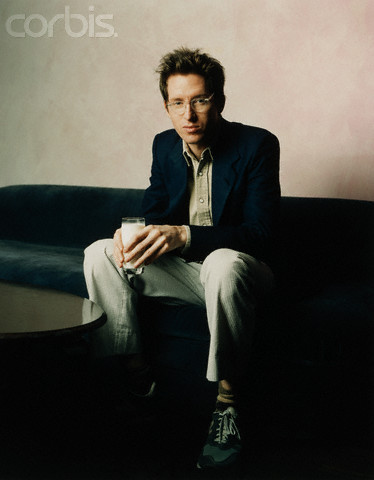The image captures a white middle-aged man sitting on a green fabric sofa in an indoor setting. He has short, spiked brown hair and is wearing frameless glasses, which complement his serious expression. Dressed in a dark-colored suit jacket over a beige shirt with the top button undone, he pairs this outfit with light-colored trousers. His ensemble is further detailed by brown socks and dark-colored trainers with white laces. The man is holding a full glass of milk in his hand. In front of him, the corner of a round, dark-colored table is visible. The backdrop behind the sofa is light-colored, and in the top left corner of the image, the watermark "Corbis" is faintly displayed.